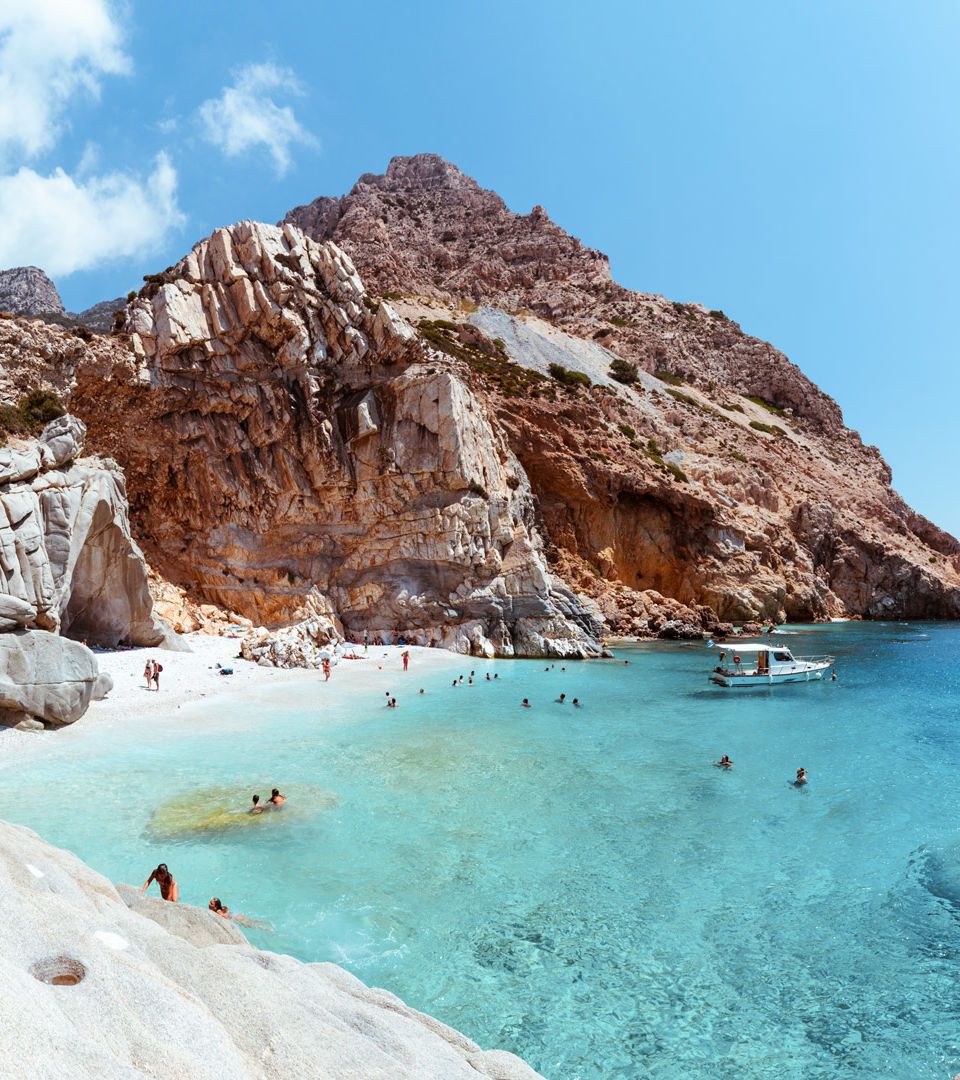The photograph captures a picturesque cove with crystal-clear, light blue water revealing the ocean floor's shallow, sandy bottom. Numerous people are swimming and enjoying the pristine, white sand beach, which appears only accessible by boat due to the surrounding steep, rocky cliffs that encircle the area. A white boat, positioned on the right side and facing away from the shore, adds to the idyllic scene. The cove is nestled within a contrasting arid, desert-like landscape, imparting an intriguing juxtaposition between the serene water and the rugged, dry cliffs. The photograph is taken from a slight elevation, likely from a rocky vantage point, providing a splendid view of the entire scene.